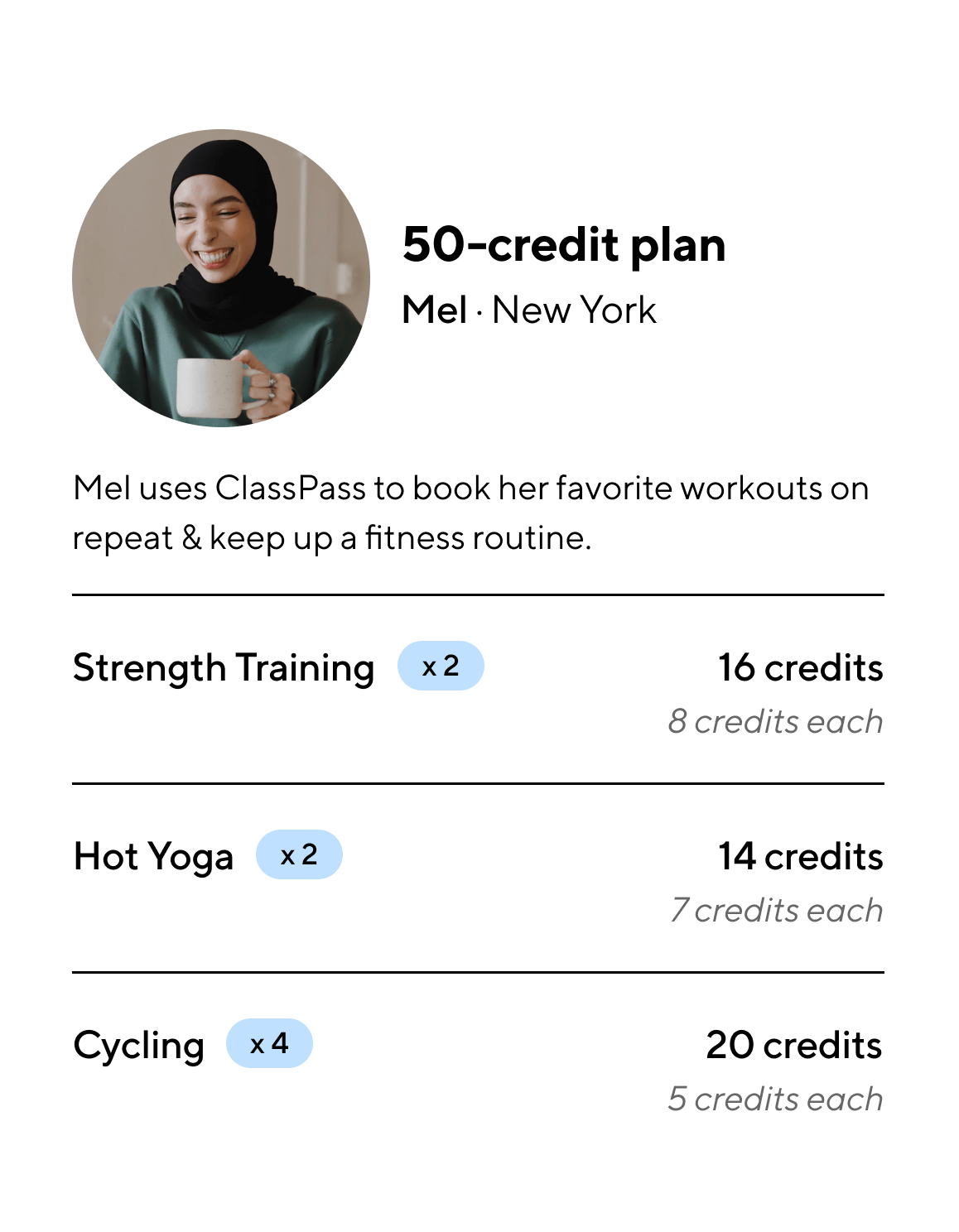The image displays an app interface showcasing a "50 Credit Plan" for a user named Mel from New York. At the top, there is a photograph of a smiling Middle Eastern or Arabic woman who is wearing a green satin shirt and a black hijab, and holding a coffee cup. Below her image, a description reads: "Mel uses ClassPass to book her favorite workouts on repeat and keep up a fitness routine."

Further down, the app details specific workout options that Mel has selected:
- Strength Training: 2 sessions for a total of 16 credits (8 credits each)
- Hot Yoga: 2 sessions for a total of 14 credits (7 credits each)
- Cycling: 4 sessions for a total of 20 credits (5 credits each)

The bottom section indicates that this interface may be part of a workout plan or an advertisement for a fitness app or program like ClassPass.